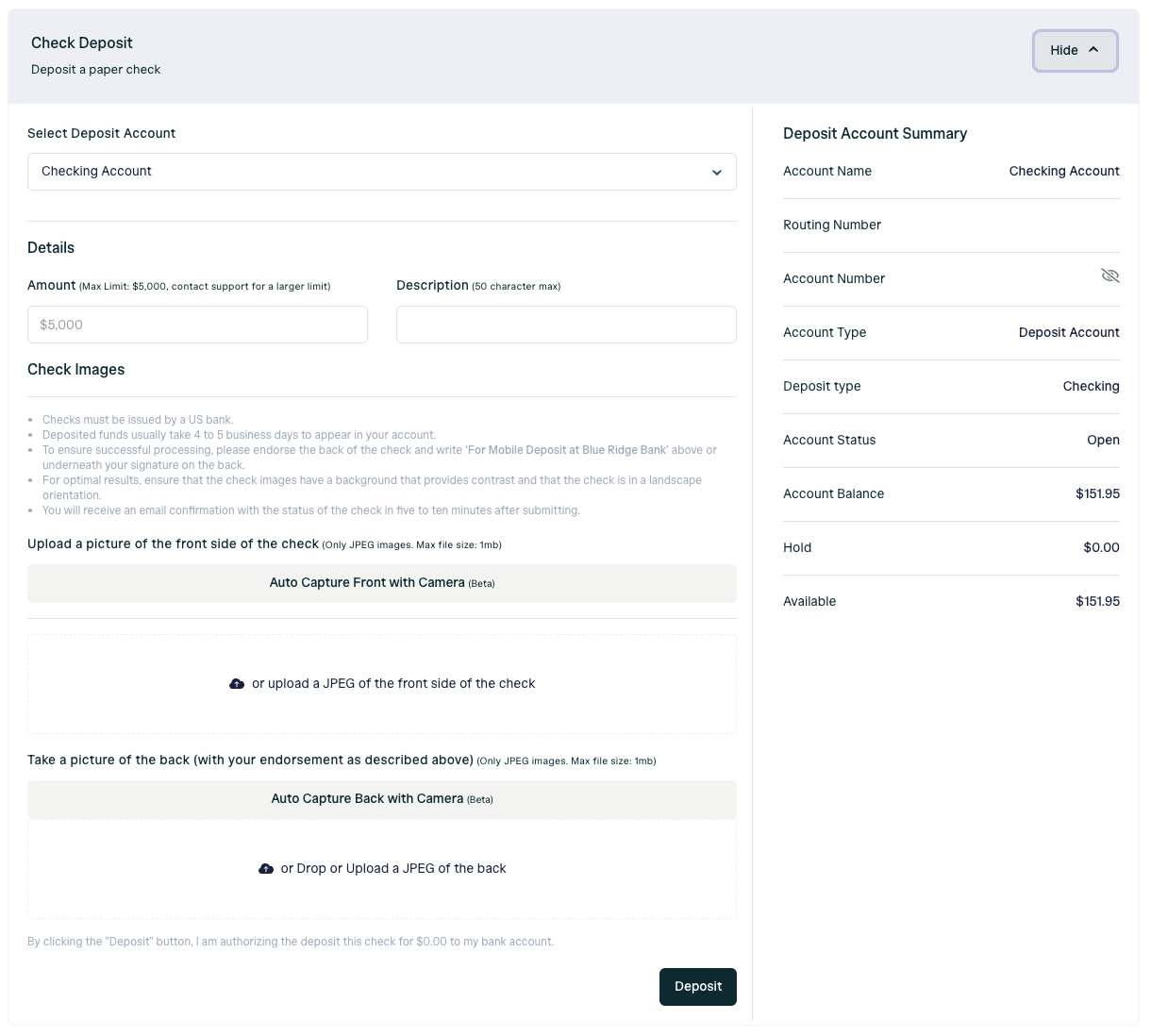**Image Description: Detailed Online Check Deposit Interface**

The image depicts an online interface for depositing a check. The background is white, providing a clean and clear presentation of the options and details.

### Header:
- **Text at the Top:** "Check Deposit"
- **Subtext:** "Deposit or Pay for Check"
- **Top-Right Corner Button:** "Hide"

### Account Selection:
- **Heading:** "Select Deposit Account"
- **Current Selection:** "Checking Account"
- **Drop-Down Arrow:** Allows the user to choose different accounts.

### Details Section:
- **Text Heading:** "Details"
- **Amount Field:** Blank, with a maximum limit of up to $5,000.
- **Description Box:** Available but currently empty.

### Check Images Section:
This section provides detailed instructions and options for uploading check images.
- **Instructional Text:**
  - "Checks must be issued by U.S. Bank. Deposited funds usually take 4-5 business days to appear in your account."
  - "To ensure successful processing, please endorse the back of the check and write 'For Mobile Deposit at Blue Ridge Bank' above or underneath your signature on the back."
  - "For optimal results, ensure that the check images have a background that provides contrast and that the check is in a landscape orientation."
  - "You will receive an email confirmation with the status of the check in 5-10 minutes after submitting."
- **Image Upload Options:**
  - **Front Side Upload Option:**
    - Button: "Auto Capture Front with Camera"
    - Option: Upload a JPEG of the front side of the check.
  - **Back Side Upload Option:**
    - Instruction: "Take a picture of the back with your endorsement as described above."
    - Button: "Auto Capture Back with Camera"
    - Option: Upload a JPEG of the back.

### Deposit Account Summary:
This section summarizes the deposit account being used.
- **Account Name:** "Checking Account"
- **Routing Number:** Unlisted
- **Account Number:** Unlisted
- **Account Type:** "Deposit Account"
- **Deposit Type:** "Checking Account"
- **Status:** "Open"
- **Account Balance:** $151.95
- **Hold:** $0.00
- **Available Balance:** $151.95

This detailed caption provides a comprehensive overview of the check deposit process and options available within the online interface.